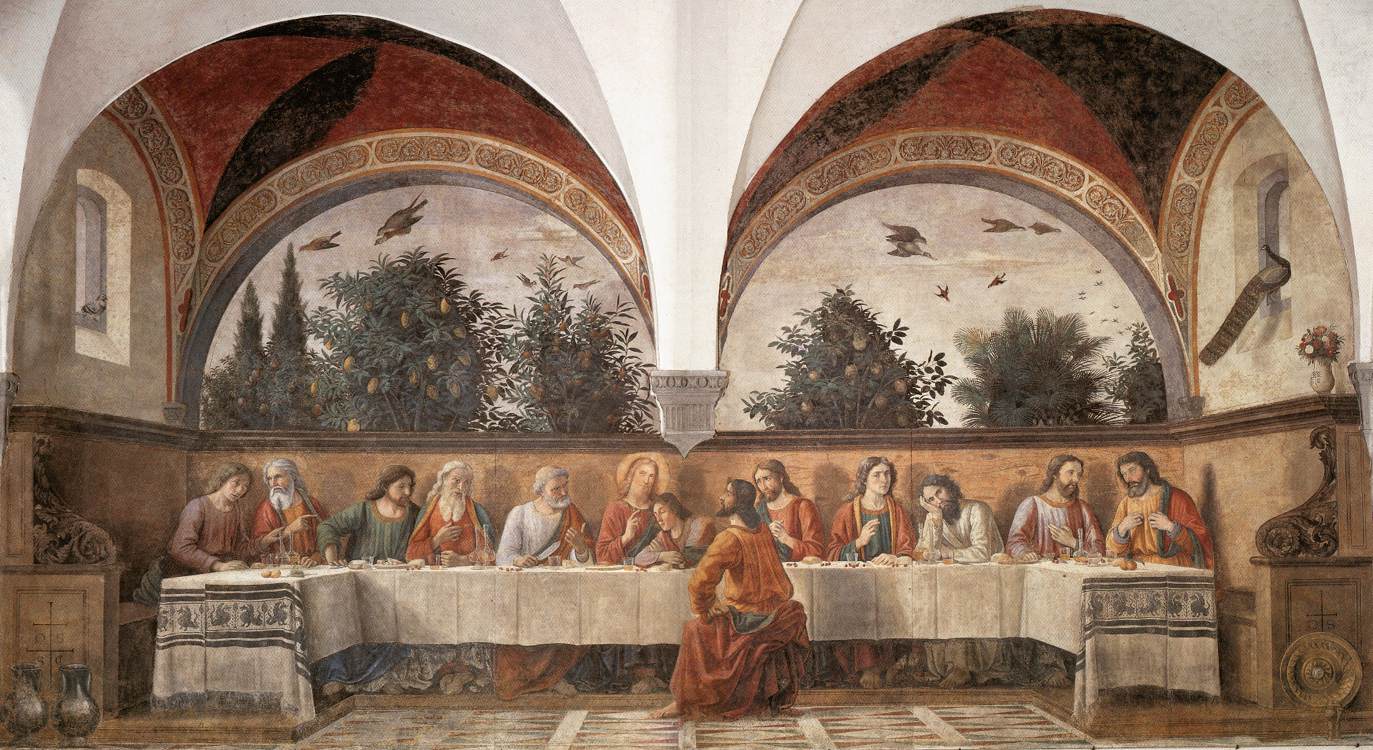This exquisitely detailed painting portrays a rendition of the Last Supper, featuring a wide rectangular canvas that captures several people seated around an elongated table. The table, extending mostly from left to right with a slight inward curve at the ends, is adorned with an off-white tablecloth with intricate blue patterns. At the center sits a man donning bright orange and red attire, indicative of Jesus, offering a focal point amidst the gathering. The individuals, predominantly men though some women are present, are all clad in ornate, thick gowns in hues of orange, green, gold, pink, and white. Many have beards, ranging in age from younger to older, some engaging in conversation and gestures, while others look contemplative. The backdrop of this lavish indoor setting showcases a high, intricately decorated ceiling with white, red, and black details, punctuated by two semi-circular windows revealing an outdoor scene with birds soaring over lush greenery. Plates of food and glasses of wine are interspersed around the table, enhancing the sacred and communal atmosphere captured in this vibrant, richly toned masterpiece.